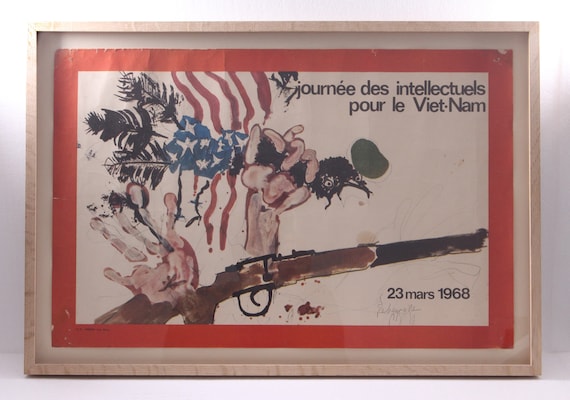This framed piece of art from March 23, 1968, titled in French "Journée des Intellectuels pour le Vietnam," serves as a poignant memento from the Vietnam War era with its haunting imagery and intricate details. The artwork features a background of white with black leaves, overshadowed by a distressed American flag consisting of red and white stripes and a blue square dotted with white stars. Central to the picture are two handprints: one pink handprint clutching an indistinct object, and another hand modeled with a finger seemingly severed, holding a brown and black shotgun, implying a violent encounter. The gun appears to have been recently used, as red marks suggest blood is pooling beneath a bird-like shape. Additional visual narratives within the frame include pencil drawings that add depth to the painted elements. The piece, encased in a wooden frame that resembles a shadow box, merges its evocative painted and penciled details to express a disturbing snapshot of conflict and loss, annotated with the historical date and French text.